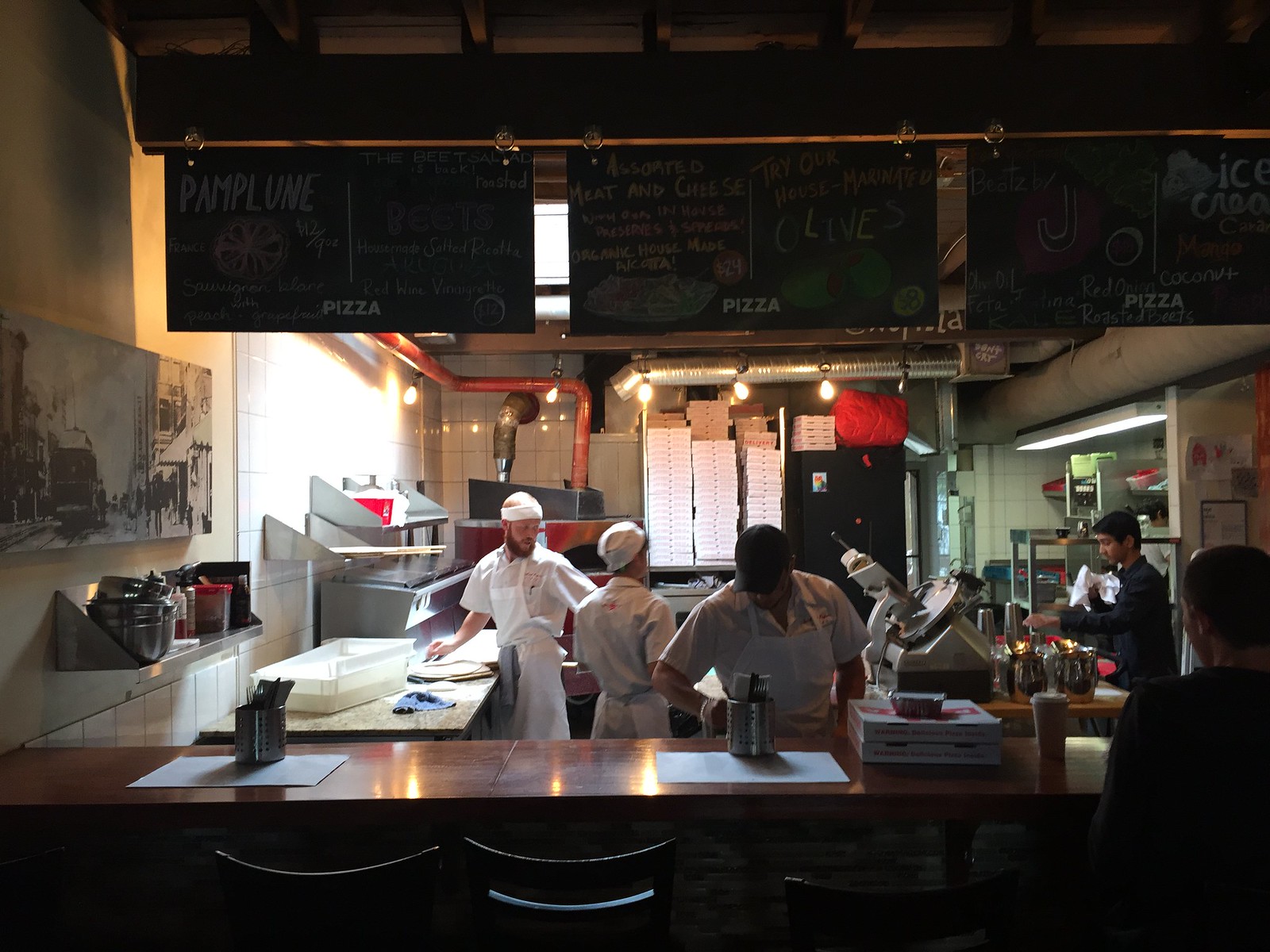The image showcases a dimly lit, behind-the-scenes look at a bustling diner, focusing primarily on its kitchen area, where takeout pizzas are prepared. The central figures are three chefs, all dressed in white shirts, aprons, and hair covers—one sporting a headband, another a hat, and the third a black cap. They are busily crafting pizzas, with one chef rolling out dough on a wooden countertop. The kitchen backdrop is filled with a myriad of pizza boxes and essential kitchen tools, including a meat cutter.

In addition to the chefs, the photo includes two individuals in black attire who appear to be customers, heading towards the counter to place their orders. The seating area in the foreground has three chairs, and above, the dimly illuminated menu board lists various pizza options and specials. The left side of the menu features a drawing of a pizza with the word "Pamploon," while the center section promotes their house-marinated olives, assorted meats, and organic house-made pizzas. On the right, unique offerings like "Beets by J-O" and "Coconut Pizza with Red Onions and Roasted Beef" are advertised. Red pipes also sporadically accent the dark color scheme of the overall setting.